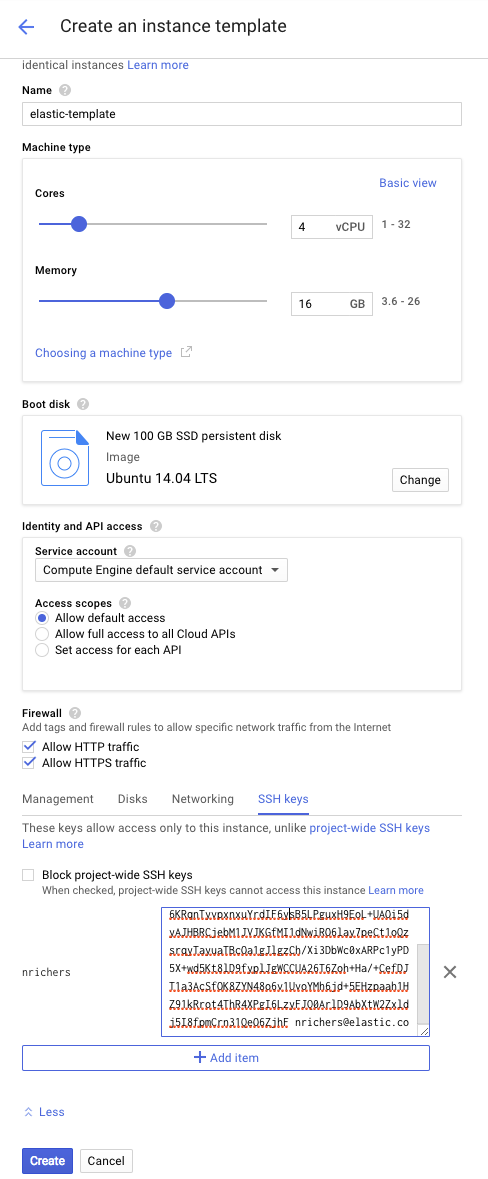The image depicts a user interface for creating an instance template, likely within a cloud computing platform. At the top, there's a blue "Learn More" button that users can click for additional information. The interface includes a section labeled "Name" with a text box, which has been filled out with the name "Classic Template."

Below the name section, there are options to select the machine type. This is done via two sliders, one for adjusting the number of cores and the other for altering memory, each marked by blue dots. Beneath the sliders, in smaller print, there's a prompt guiding users on "Choosing a machine type."

Further down, there's a section labeled "Boot Disk," accompanied by a blue disk icon and a brief description. The next section is for "Identity and API Access," which provides a brief explanation inside a bordered box. This is followed by a "Firewall" section where two options – "Allow HTTP traffic" and "Allow HTTPS traffic" – are listed with checkboxes next to them; both checkboxes are ticked.

At the bottom, additional management options are provided under tabs labeled "Management," "Disks," "Networking," and "SSH Keys," the latter highlighted in blue. There's an explanation about the keys, but some text appears distorted in red and black, making it difficult to read.

Finally, at the very bottom of the interface, there are two buttons: a blue "Create" button and a "Cancel" button.